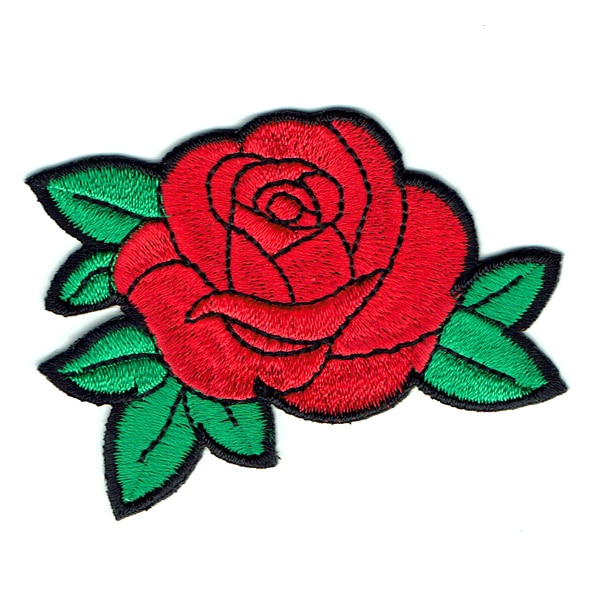The image showcases an embroidered patch against a solid white background, featuring a vivid red rose surrounded by green leaves. This patch, meticulously crafted from fabric and thread, is outlined with a prominent black border. The rose and leaves also include intricate black line details, with the leaves having a central thin black line. This versatile patch, which could be sewn or ironed onto garments, such as a college football team's jersey or a band member's uniform, highlights the textured threads and stitch directions used to create the detailed floral design.